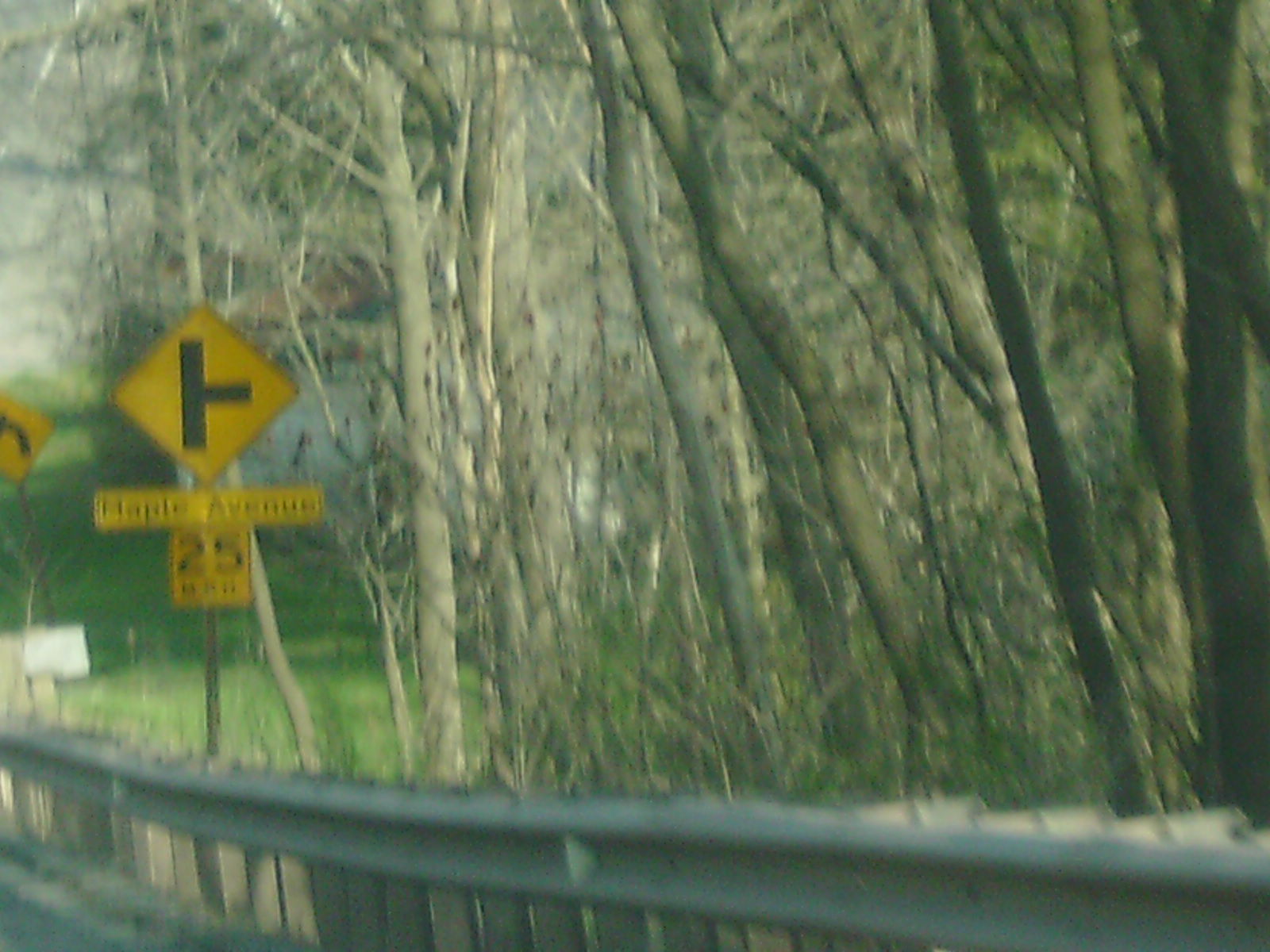A color photograph, slightly blurred and with a greenish-yellow tint, appears to be taken from inside a car, likely from the passenger's window. The image captures a road or walkway alongside a woodland area with tall, leafless trees that have slender, gray trunks and some light filtering through. To the right, there is a silver guardrail supported by brown wooden posts running across the middle to the bottom left of the image. Multiple street signs are visible, including a larger yellow diamond-shaped sign indicating a T-intersection for Maple Avenue with a smaller rectangular sign below it showing a speed limit of 25 miles per hour. In the far left, there's another yellow diamond-shaped sign, likely indicating a curve ahead. The scene is set in daylight, possibly around noon based on the shadows. A white building or house is faintly visible in the distance, adding to the detailed, albeit blurry, depiction of this roadside landscape.